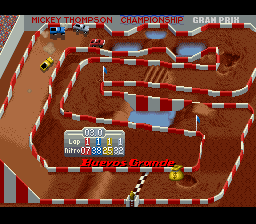The image depicts a vibrant scene from a video game showcasing an exhilarating car race. The backdrop prominently features the title "Mickey Thompson Championship," indicating a prestigious racing event. The racetrack appears to be a miniature, model version, adding a whimsical touch to the setting. Four vividly colored vehicles—a yellow, a blue, a light blue, and a red car—are seen competing fiercely on the track.

The racing teams' standings are displayed on signage, providing scores and contributing to the competitive atmosphere. The event is named "Juegos Grande," which translates to "Grand Games," and this title is boldly presented along with an illustrative symbol of a bag of gold, suggesting a significant reward or prize.

The racetrack itself is bordered by red and white stripes that resemble a candy cane motif, enhancing the playful and festive ambiance. The track layout is detailed within what appears to be a cardboard box, adding a layer of charm to the scene. Additionally, the track surface features earth-toned dirt, adding a realistic texture to the otherwise fantastical setting where the cars are racing.